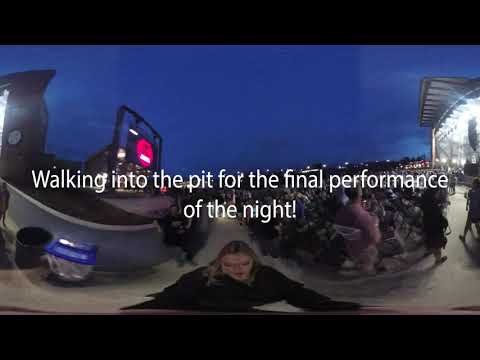The distorted, blurry image, possibly a panoramic shot, captures a nighttime outdoor concert festival. At the bottom center of the frame is a person with long blonde hair, most likely taking the photo. This individual, distorted and squashed in appearance due to the image quality, wears a black shirt. Surrounding this central figure, the scene reveals an audience seated in chairs, all facing a brightly lit stage. This gathering, implied by the caption "walking into the pit for the final performance of the night," suggests the anticipation of a significant event. The sky above is dark, contrasting with the vibrant stage lighting and the modern, glass-windowed building towards the left, which features a red circle traffic sign. The overall ambiance is lively, with people scattered across the scene, enhancing the festival atmosphere.